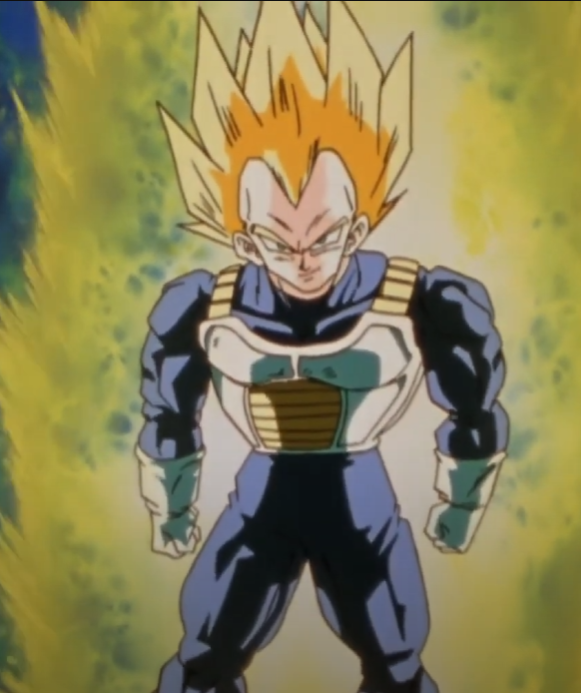The image depicts a highly detailed and nostalgic animation cell from the classic 1990s anime, Dragon Ball Z. The central character is Vegeta, the Saiyan Prince, mid-transformation into his Super Saiyan form. Vegeta's signature spiky blonde hair is prominently displayed, with a brilliant golden aura surrounding him. His muscular build is accentuated by his blue, skin-tight bodysuit, which covers him from neck to feet. Over this, he wears a distinctive white battle armor with yellow accents on the straps and midsection, and white gloves that extend past his wrists.

Vegeta's pose is dynamic; his arms are positioned side by side, fists clenched, exuding power and readiness for combat. He stares directly at the viewer with large, intense anime-style eyes and a characteristic arrogant smirk, underlining his confident and formidable nature. The background is almost indiscernible, dominated by a striking flash in neon green, white, and yellow hues, adding to the dramatic atmosphere of the scene. This vibrant depiction stays true to the original animation style, evoking a sense of nostalgia while showcasing the iconic Super Saiyan transformation.